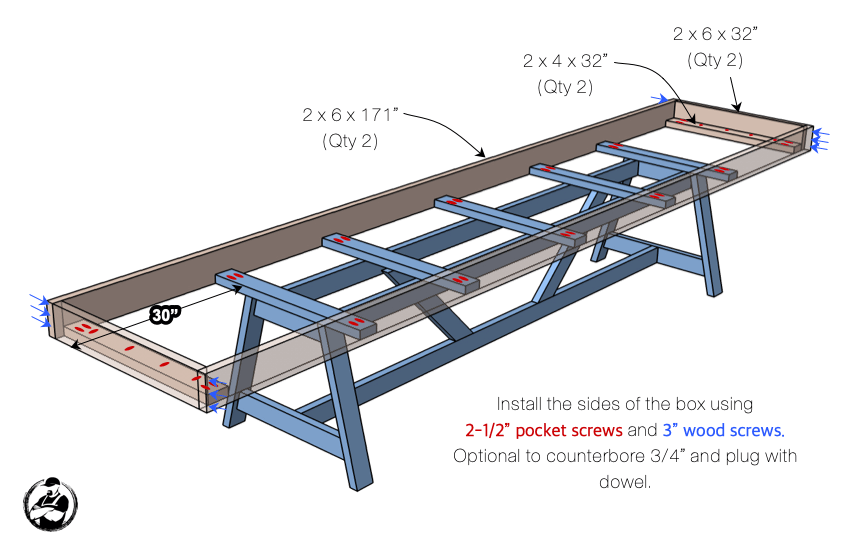The image is a detailed instructional diagram typically used for assembling furniture. It prominently features a box-like structure with dimensions similar to a table. The box measures approximately 2 inches by 6 inches by 171 inches, with an alternative measurement of 2 inches by 4 inches by 32 inches for additional parts. The diagram shows a long surface on top supported by a leg system and highlights the construction using pocket screws and wood screws. Specifically, it instructs to "install the sides of the box using 2 1/2 inch pocket screws and 3 inch wood screws," with an optional step to "counterbore 3/4 inch and plug with a dowel." Blue arrows indicate where screws should be placed. The diagram also shows a wooden frame positioned on a sawhorse-like device, with the long and shorter wooden boards arranged perpendicularly to form the structure. The illustration is set against a white background with this detailed text included.